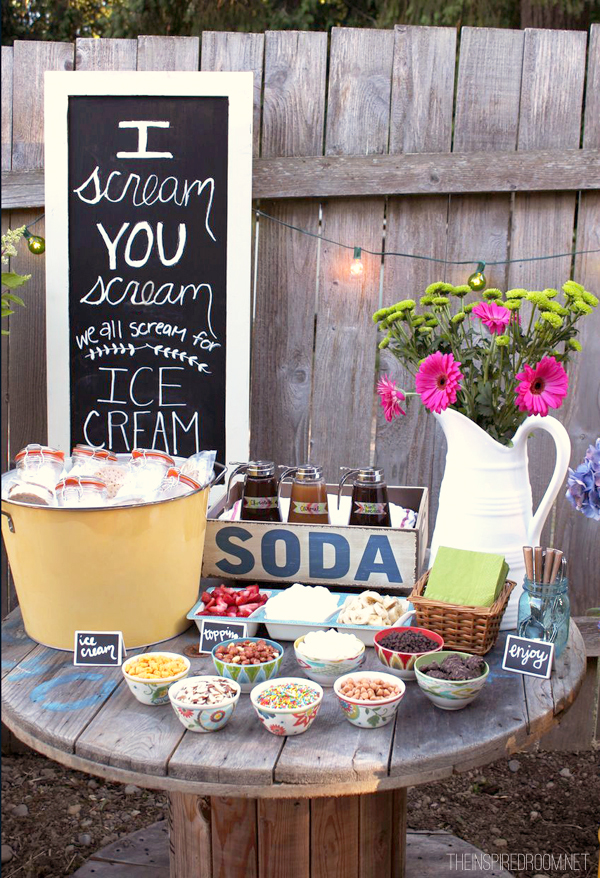The image displays a charming outdoor dessert station set against a weathered clapboard fence. At the heart of this setup is a circular wooden table fashioned from an old spool. Atop the table is a playful chalkboard sign that reads, "I scream, you scream, we all scream for ice cream." Dominating the left side of the table is a large yellow enamel bucket filled with ice and multiple mason jars, likely containing ice cream. Beside it, an old wooden soda crate holds an array of syrup dispensers for caramel and chocolate toppings. The center of the table features a platter and eight small bowls filled with various toppings, including M&M's, nuts, coconut, and chocolate chips. To the right, there is a basket with green napkins and a blue mason jar filled with wooden-handled spoons. A tall white enamel vase behind the napkins holds a bouquet of pink gerbera daisies and yellow wildflowers, adding a splash of color to the rustic display. The table stands on bare dirt, enhancing its rustic charm.